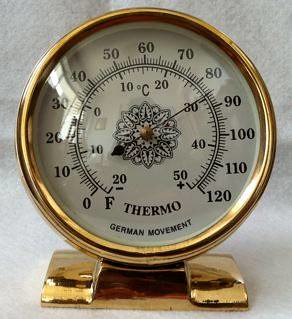This color photograph features a round, gold-plated thermometer encased in glass. The face of the thermometer displays both Fahrenheit and Celsius scales, with Fahrenheit ranging from 0 to 120 degrees and Celsius from -20 to 50 degrees. At the bottom of the face, the words "Thermo" and "German Movement" are inscribed. The numerals and the pointer, placed centrally on the dial, are black, providing a sharp contrast for easy readability. The middle of the faceplate is adorned with an intricate floral pattern, adding an aesthetic touch to the instrument. The thermometer, set in a gold base and protected by a glass cover, combines functionality with elegant design.